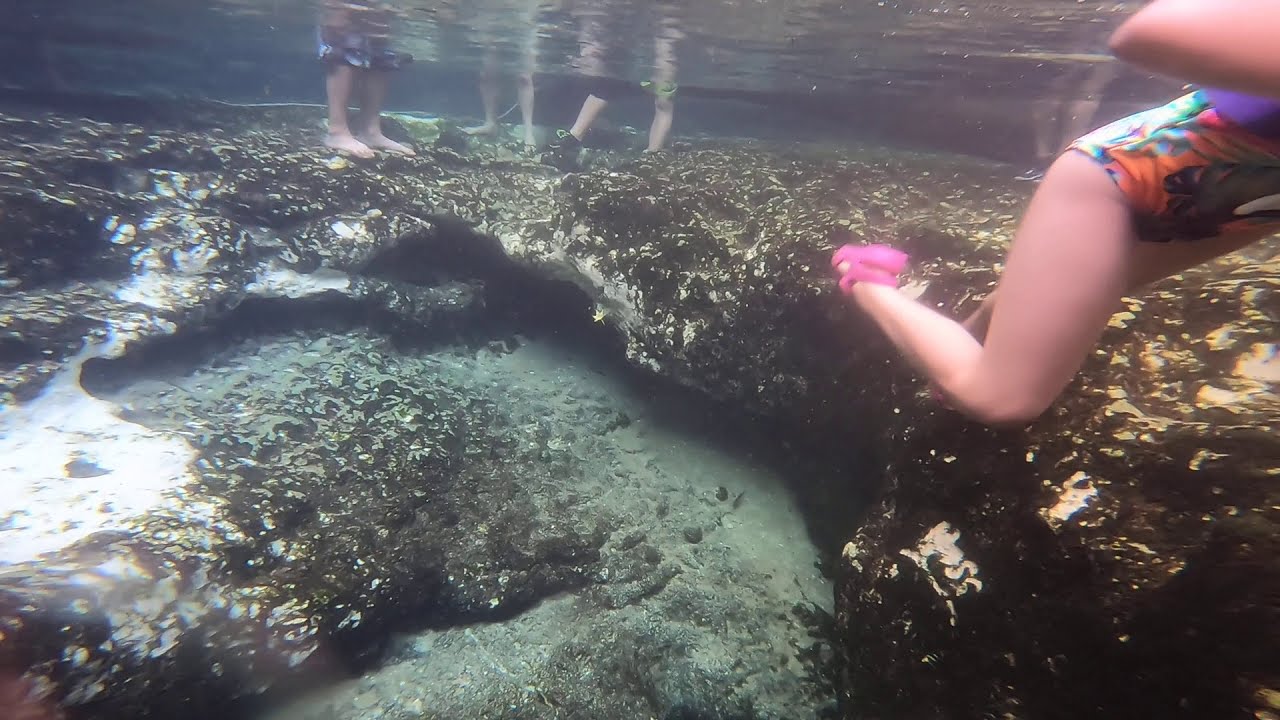This underwater photograph captures a serene and playful scene near a shoreline, where a few children frolic among natural rock formations. Dominating the right side of the image, a girl is perched on a rock, with her cropped body showing from chest to legs. She wears pink sandals and a vibrant one-piece swimsuit featuring a tie-dye pattern of orange and green. The image also includes the partially visible legs and feet of three other children, submerged up to their knees, standing on the uneven, algae-speckled rock surface. The rocky seabed is dotted with areas of sand, and though the water is shallow, the top appears wavy from below, reflecting the light filtering through. No sea grass, moss, or marine creatures are visible, highlighting the natural simplicity of the setting.